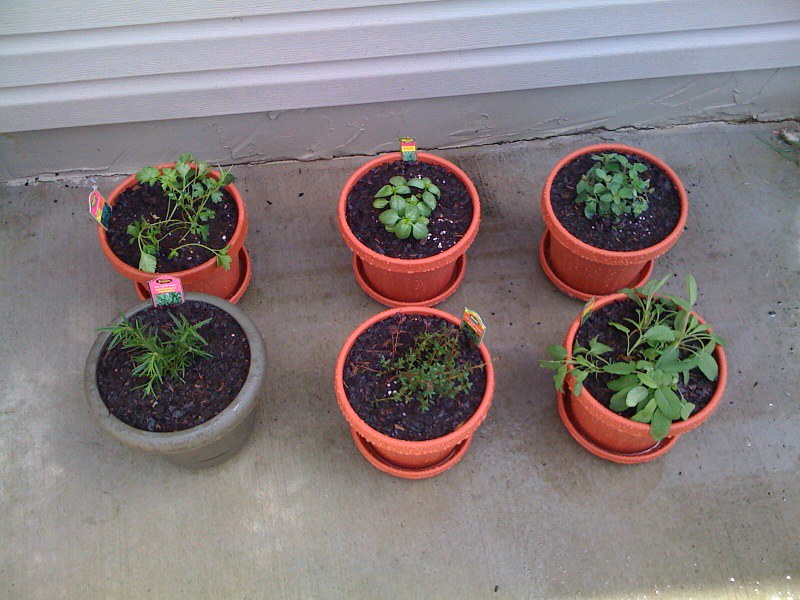This color photograph captures an overhead view of six potted plants arranged neatly on a concrete surface, flanked by a white building wall. The pots are organized in two rows of three, with five of them being an orange-red clay color, each accompanied by a matching red saucer, while the sixth pot, situated at the bottom left, is a distinct gray stoneware planter. Each pot is filled with dark, rich soil, from which various types of green, leafy plants emerge. These plants differ in appearance, with some having tall, long, and pointy leaves, while others exhibit more clustered foliage. Notably, an identification tag protrudes from the soil in one of the pots, though its writing is illegible. The photograph is straightforward, emphasizing the serene, leafy arrangement on what looks like an exterior patio devoid of people, animals, or mechanical objects.